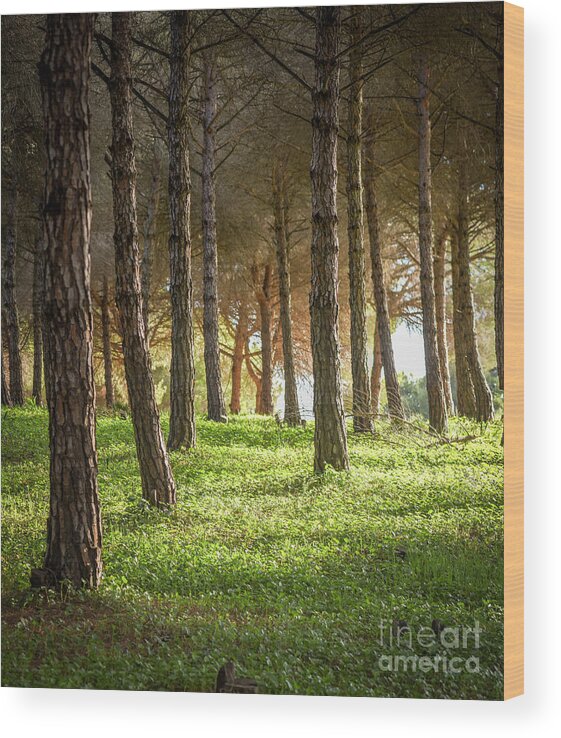This image is a detailed photograph mounted on a rectangular wooden board, which has a natural brown texture visible from its thin side view. The photograph, capturing a forest scene, features numerous slender tree trunks extending skyward, mostly devoid of leaves, creating an organized yet dense appearance. The forest floor is lush with green grass interspersed with some white wildflowers, and the sunlight filtering through the trees hints at either a sunrise or sunset, giving the scene a warm, glowing ambiance. The background shows a mix of slightly blurry trees, suggesting depth and distance within the forest. Positioned at the bottom right corner, a watermark reads "Fine Art America" against the green grass.